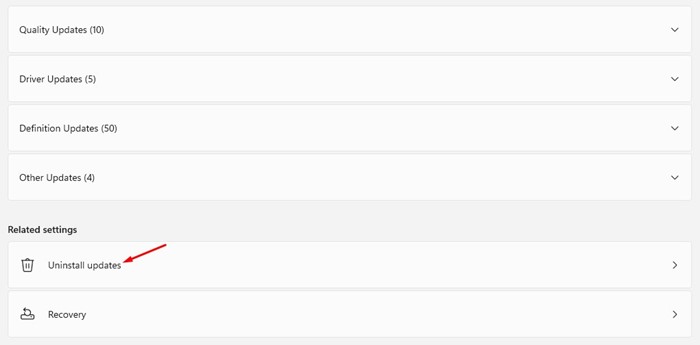The image is a screenshot of a website featuring a minimalistic design with a predominantly gray background and horizontal white bars, each containing different topics. The first bar is labeled "Quality Updates (10)" and includes a down arrow on the far right, suggesting it can be expanded to reveal more information. The subsequent bars are labeled "Driver Updates (5)", "Definition Updates (50)", and "Other Updates (4)", each similarly featuring a down arrow for additional options. Heading the section is a title reading "Related Settings". Below this title are two white bars: the first features an icon of a trash can and the text "Uninstall Updates", accompanied by a red arrow pointing to it, indicating its importance. The second bar displays an obscure flat box symbol with a circle, likely representing a computer or system, and is labeled "Recovery".